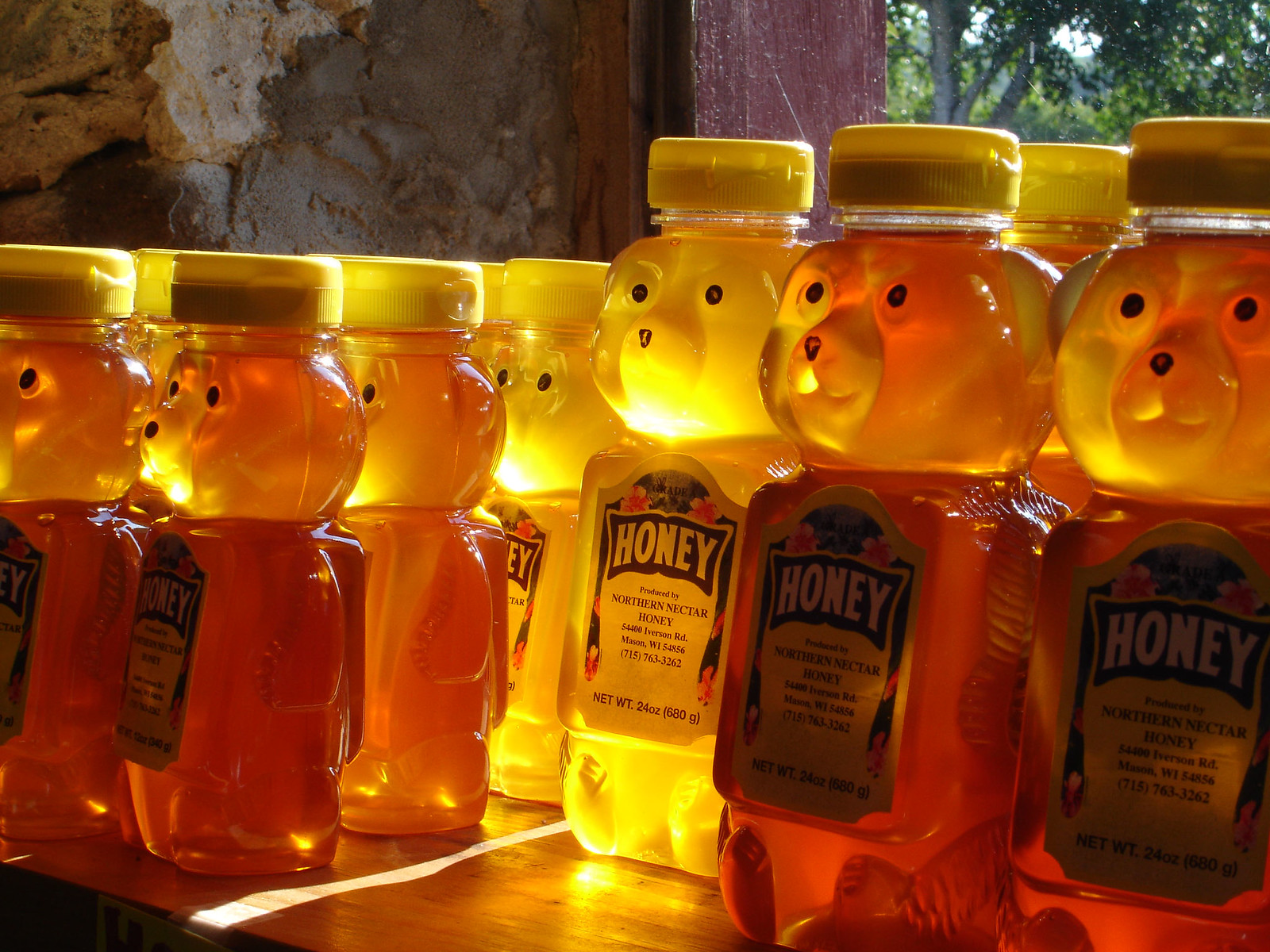This close-up photograph showcases at least twenty honey bear jars, neatly lined up on a wooden table in front of a rustic stone wall. Each jar, made of plastic, is shaped like an adorable bear, complete with 3D extrusions for eyes, nose, arms, and feet. They feature black eyes, a snout, and each has a yellow twist-off cap. Some of the honey inside is darker, while others are lighter, ranging from yellowish to reddish-brown hues, illuminated by sunlight filtering through a nearby window with a maroon wooden sill. Outside the window, a large tree with dark green leaves is visible against a blue sky, suggesting a sunny day. The bear-shaped containers have rectangular labels on their chests that say "Honey," along with additional text that includes "northern nectar honey," although some details are difficult to read. The setting is charming with the unevenly plastered stone wall adding a cozy, natural backdrop.